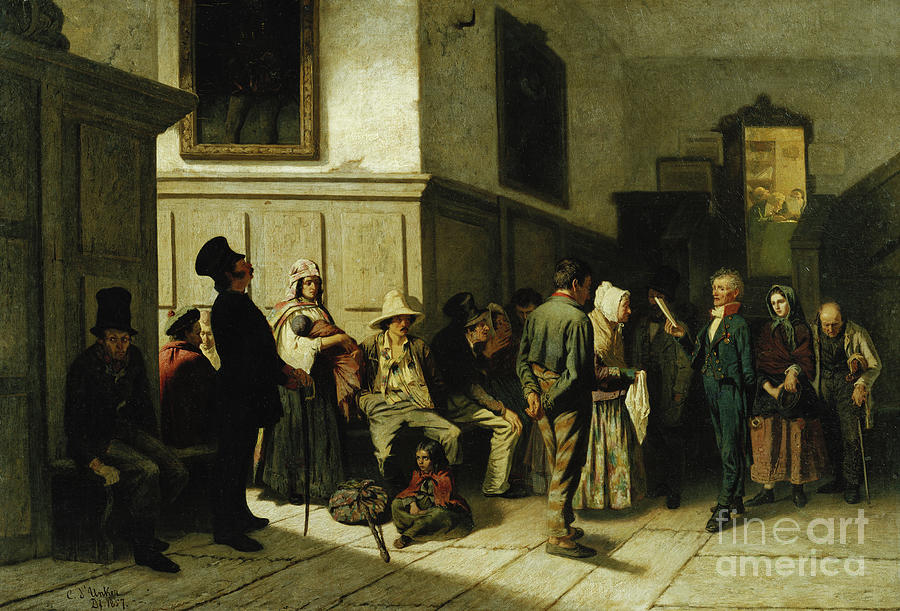This highly realistic painting, appearing to date back to older England, presents a scene of stark social contrast within a grand, opulent indoor setting. The room features remarkably high ceilings, likely around 20 feet tall, and is adorned with wood-paneled walls, large paintings, and an ornate mirror in the background. In the bottom right corner, the text "Fine Art America" is subtly inscribed in white lettering.

At the center of the scene, an authoritative figure clad in formal attire — a blue jacket and matching pants with a white undershirt — holds a piece of paper, seemingly reading aloud or directing the gathered assembly. To his left stand several well-dressed individuals, likely representing the upper echelons of society, while on his right and in the background are groups of less fortunate people.

Notably, in one corner, a boy in worn clothing sits on the floor beside a sack tied to a stick. Nearby, an elderly man leans on a cane, with a girl beside him. Among the diverse crowd, an elderly woman stands in front of the official, possibly awaiting assistance or instructions.

Other poor-looking figures are scattered throughout the room, including a woman holding a baby and several others seated on a bench along the wall. In the shadows, a man in a top hat stares intently forward, adding a somewhat eerie element to the composition. Additionally, a staircase with a golden doorway can be seen, leading to another area where a few men sit around a table, looking like the important individuals to whom the crowd might be waiting to speak.

The entire scene, set against a backdrop of beige and gray tones and a floor of large wooden planks, suggests a moment of social disparity and bureaucratic procedure, captivatingly captured in this artful depiction.